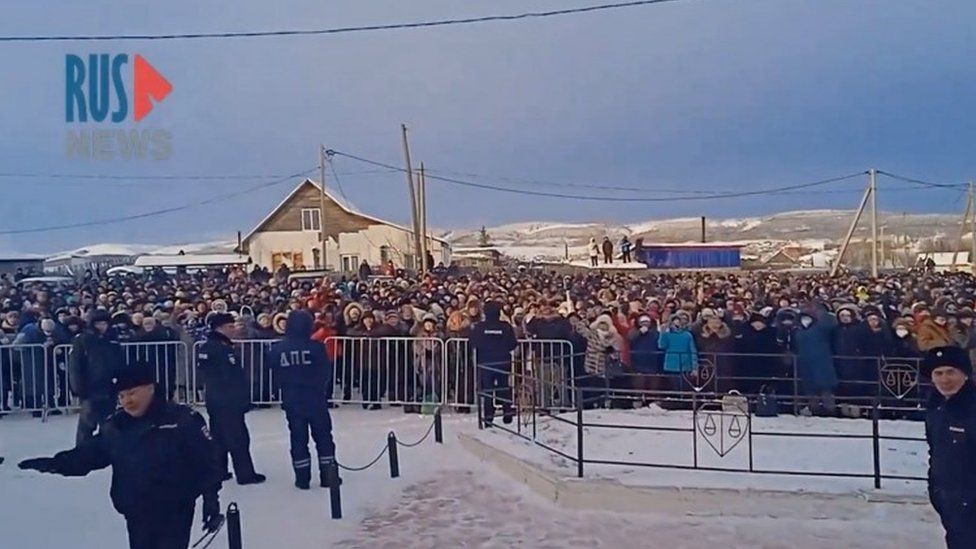In this detailed image likely depicting a newscast, the upper left corner features the RUS News logo, with "RUS" in large blue letters, a red sideways triangle, and "NEWS" in off-white. The outdoor winter scene is set against a clear blue sky. In the foreground, five or six uniformed police officers stand in the snow, clad in blue winter gear with hats or hoods, guarding an iron gating fence. Behind them, an enormous crowd of people, bundled in coats and hoods against the cold, stretches across the scene. In the background, a brown, single-story building with a white, pitched roof is visible, alongside telephone poles and wires. The image, almost twice as wide as it is tall, captures the chill of the day and the sense of tension at what might be a protest or large gathering.